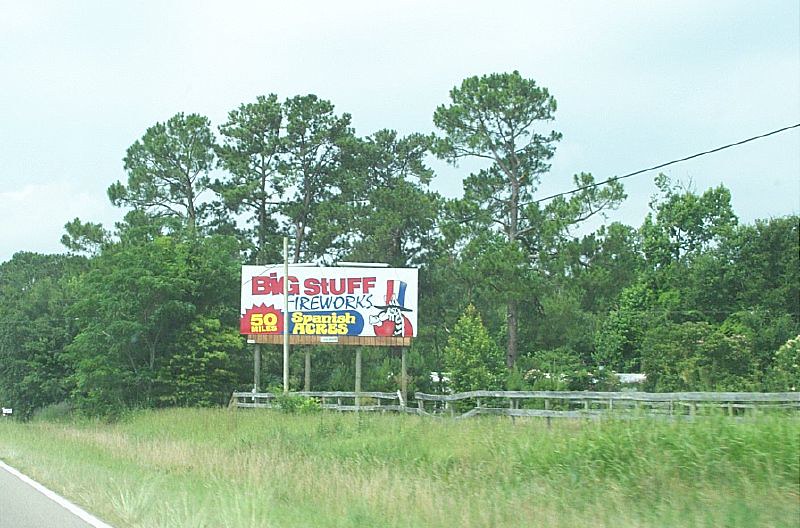The image captures a vivid outdoor scene, seemingly taken from the side of a road or possibly through a car window. The sky is a bright blue adorned with scattered white clouds, providing a picturesque backdrop that meets a dense tree line. The trees are tall, lush, and vary in shades of dark and light green, creating a full, vibrant canopy. Nestled behind the trees is a white building partially obscured by the foliage. A wooden fence, weathered and gray, runs along the right to left, partially broken at points and extending three-fourths across the image near a road’s grassy embankment visible in the bottom left corner. 

Dominating the scene is an old billboard, upheld by four large posts, featuring a mix of colorful text and graphics. Bold red letters spell out "Big Stuff" at the top, with "Fireworks" in blue underneath. In the bottom left of the sign, "50 Miles" is written in yellow amidst a red starburst pattern, while "Spanish Acres" appears in yellow with a blue circular background. The right side of the billboard displays a whimsical character, possibly a giraffe, adorned in a red outfit and a red, white, and blue striped top hat. A pole beside the billboard supports wires, adding to the intricate details of this roadside snapshot.